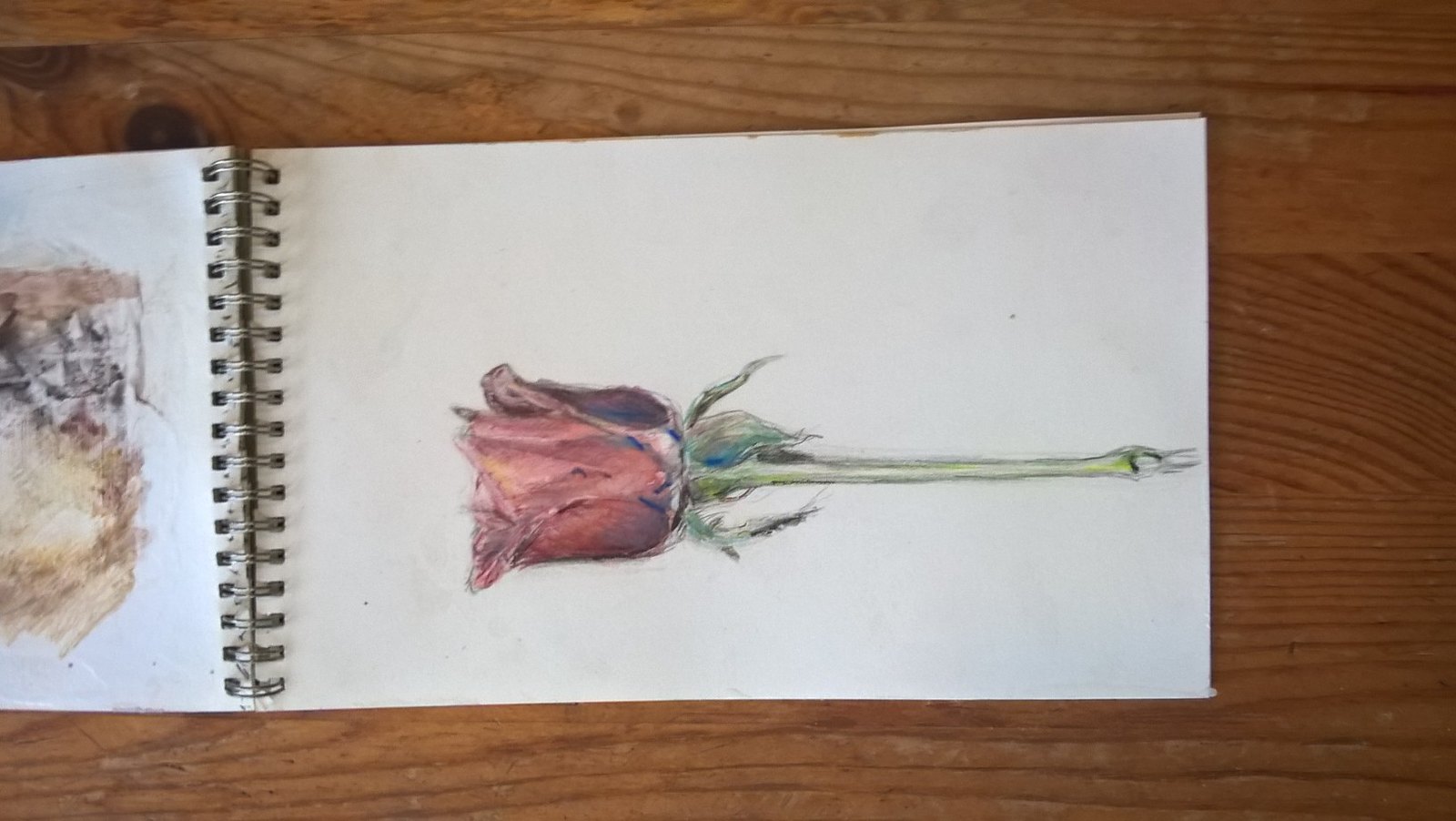The image features a sketchbook lying on a light brown hardwood surface, which could be either a table or the floor. The sketchbook is opened and positioned horizontally, with the bottom part extending to the right-hand side of the frame. The top part of the sketchbook is partially out of view, but a glimpse reveals a drawing or painting of a brown dog, rendered in colored pencil or crayon. The primary focus of the visible page is a detailed illustration of a red rose with a green stem and leaves. This rose occupies the majority of the sketchbook page and appears to be executed in a similar medium of colored pencil or crayon.